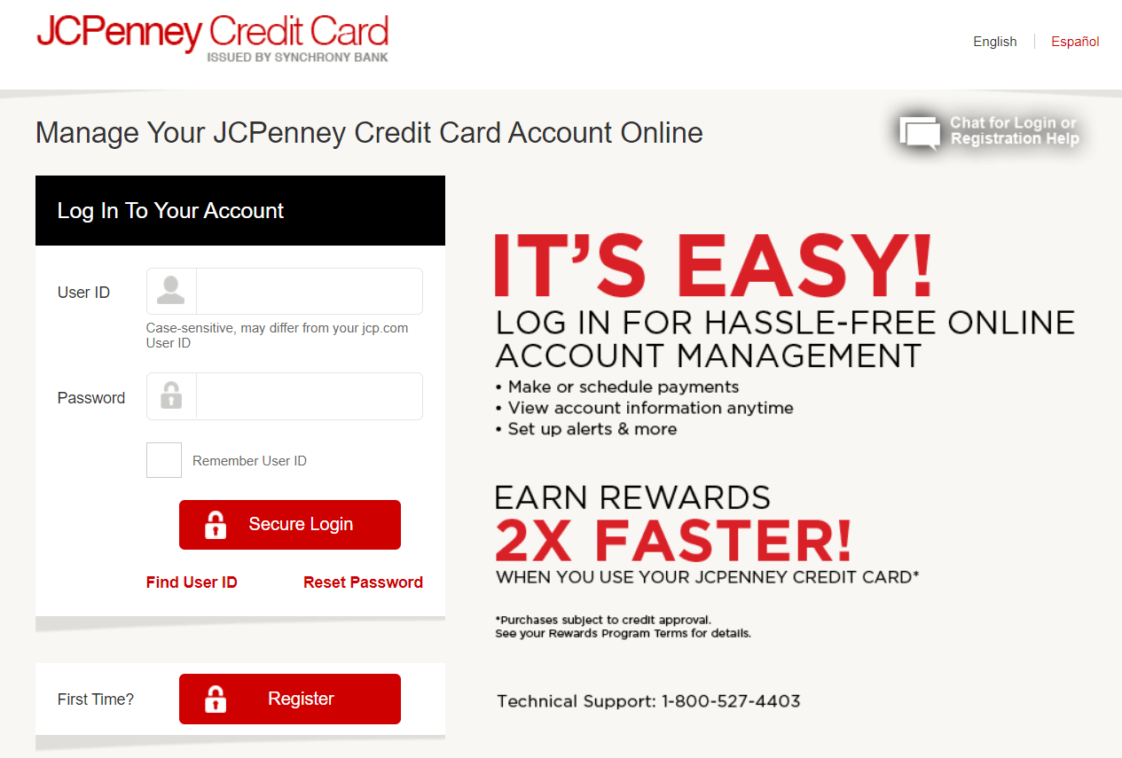This image depicts a JCPenney Credit Card login webpage, issued by Synchrony Bank. Dominating the page is a prominent header offering hassle-free online account management. Beneath the header, three main points highlight the benefits, including earning rewards twice as fast when using the JCPenney Credit Card, accompanied by an asterisk linking to terms and conditions, subject to credit approval.

Central to the page is the login section. The top area includes fields for 'User ID' and 'Password', with 'User ID' noted as case-sensitive. Below these fields, there is an option to check a box to 'Remember User ID'. Directly underneath is a prominent 'Secure Login' button to access the account. 

In case of forgotten login credentials, there are buttons labeled 'Find User ID' and 'Reset Password' for user assistance. Lower on the page, a section addressed to new users displays the question, 'First time here?' followed by a 'Register' button with a small lock icon, inviting them to register for an account.

The upper-right corner of the page features a 'Chat' button for login or registration help. Near the bottom, the page also provides a technical support contact number for further assistance. The clean layout and clear instructions ensure users can easily manage their JCPenney Credit Card accounts online.